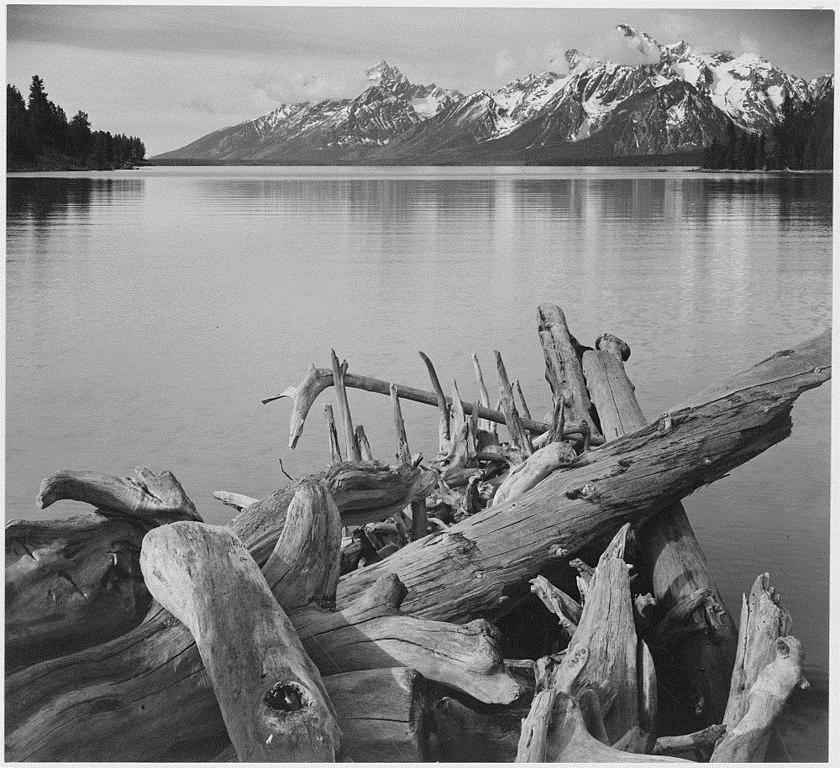A highly detailed black-and-white photograph captures a serene lakeside scene, emphasizing heavy contrasts reminiscent of an Ansel Adams piece. In the foreground, a pile of intricately intertwined driftwood of various shapes and sizes—mangled, gray, and blackened with shadows—forms a striking centerpiece. These logs range from curly to straight, broken off to thick and pointy at the top. This driftwood is set against the backdrop of a calm lake, its surface reflecting light with hints of gray and purples. 

On the left, a dense line of dark green trees, likely evergreens, rises tall and casts its stark reflection onto the water. To the right, a row of sharp, jagged mountains, dusted with snow at their peaks, fades into the gray clouds above, which appear full and heavy with rain. The sky transitions to a slightly lighter hue towards the left side, adding depth to the grayscale palette. The entire composition showcases exceptional skill in capturing contrasts and details, lending the image a sense of tranquil majesty and photorealistic precision.